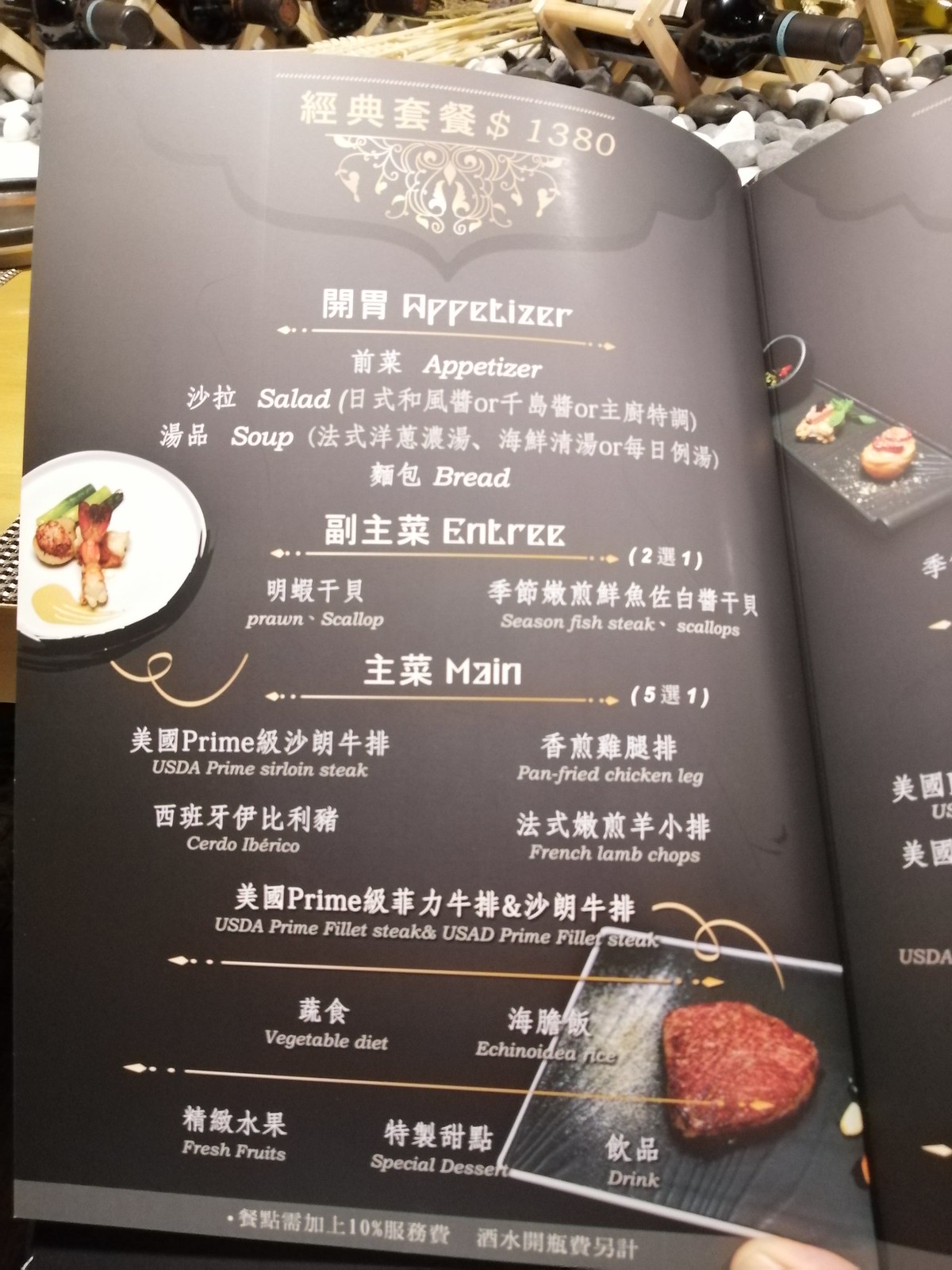In the image, we see the open menu of what appears to be a sophisticated, upscale restaurant. The menu is primarily in either Chinese or Japanese, with translations provided for each item. The menu is the main focus, occupying most of the frame, but in the background, you can glimpse a decor featuring river stones—smooth, round rocks—arranged on the table. The table itself seems to have a pine bamboo appearance, adding a natural, elegant touch to the setting.

The menu page visible in the image lists various sections such as appetizers, salads, soups, and entrées. Specific entrée options include prawns and scallops, illustrated with an image depicting two shrimps, one scallop, and a few pieces of green onion. Other entrées listed are pan-fried chicken leg, French lamb chops, cerdo iberico, USDA prime filet steak, and another similarly named steak, possibly indicating a premium selection. The menu also mentions a vegetable diet, a certain "echinolean diet," fresh fruits, special desserts, and drinks.

To the right, there's a hint of another menu page, suggesting additional selections not fully visible in this image. The overall presentation is very refined, with minimalistic and decorative plating. The setting and details reflect a high-end dining experience, emphasizing culinary artistry and sophistication.